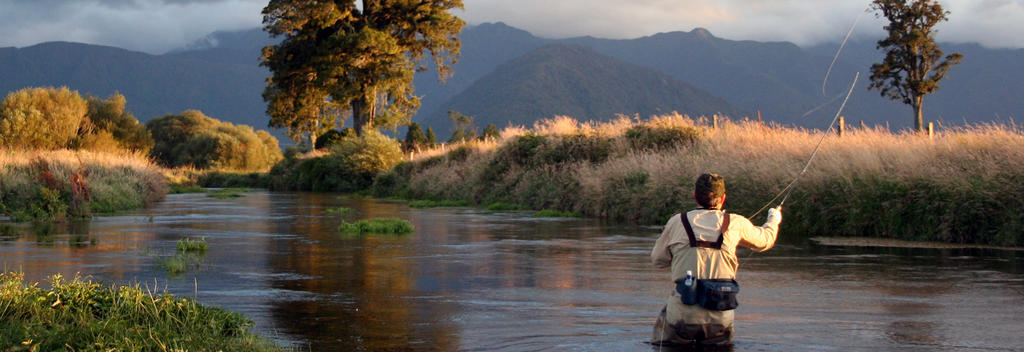This ultra-wide panoramic color photograph captures an idyllic scene of a man fly fishing alone in a calm, small river. The man's back is turned towards the camera, and he is captured mid-cast, with his fishing rod arched back and the line visible in the air. He is standing waist-deep in the dark, serene water, dressed in full waders held by suspenders and wearing a yellow shirt. A black fanny pack is strapped around his waist, pushed towards his back. The river is around 20 to 30 feet wide with patches of green vegetation dotting its course. The banks are gently sloping with a mix of dried wheatgrass, dark green elements, and sagebrush. Two deciduous trees, a large one in the center and a smaller one on the right, add to the scenic beauty. In the background, majestic hills and mountains rise under a very cloudy sky, completing the tranquil outdoor setting.